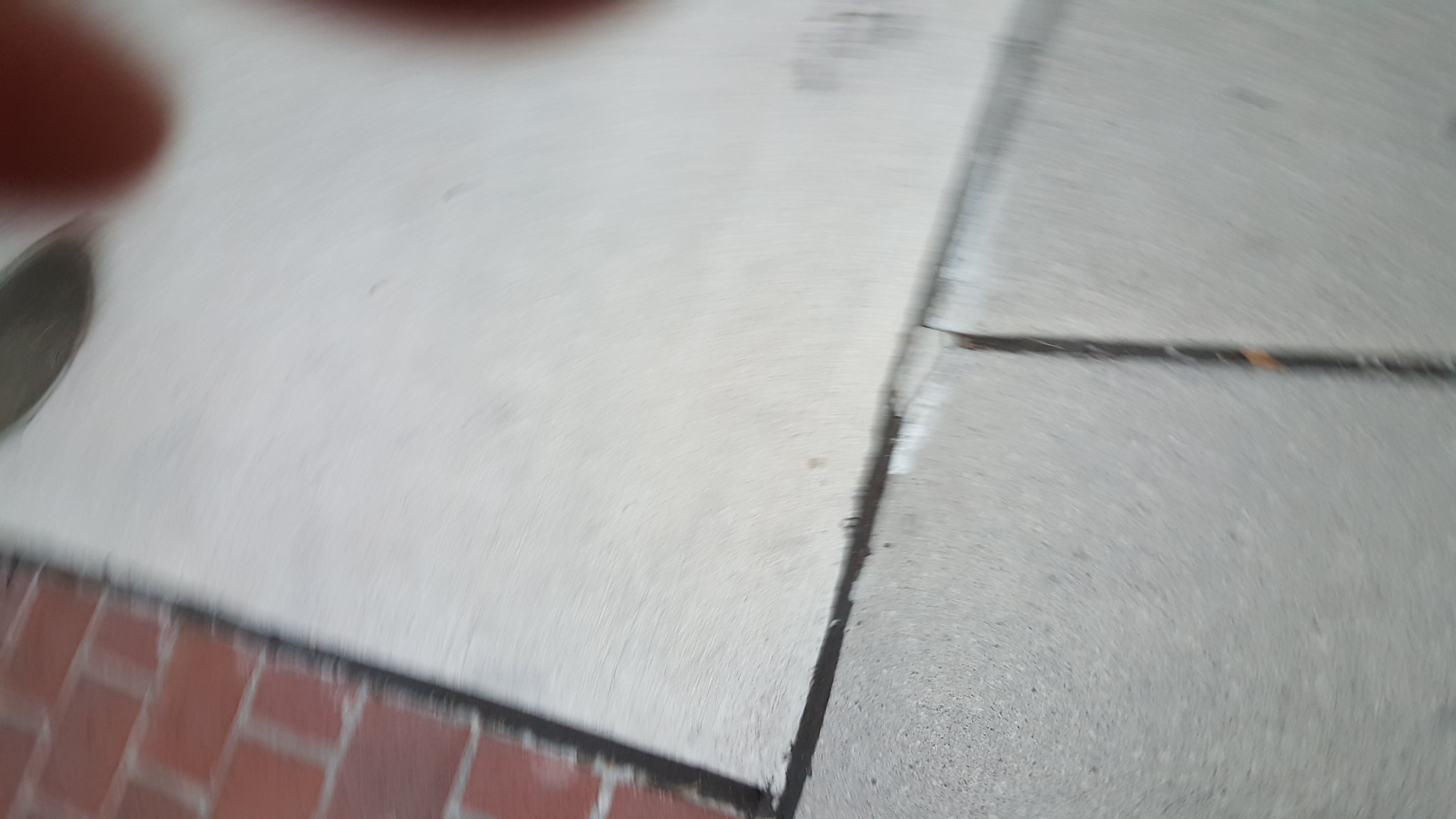This color photograph, seemingly taken with a GoPro or similar head-mounted camera, presents a somewhat blurry and close-up view, making it challenging to discern the precise subject matter. In the top left corner, blurry human fingers are partially visible, suggesting the photographer's involvement. The foreground features several white tiles or slabs that appear gray due to lighting or dust; one large tile is prominently placed from the center to the left, while two smaller tiles are situated to the right. A segment of red brick is noticeable in the bottom left corner, adding a contrasting texture to the scene. The image has a landscape orientation, being wider than it is tall. There are no writings, animals, plants, flowers, or trees present in this particular photograph.